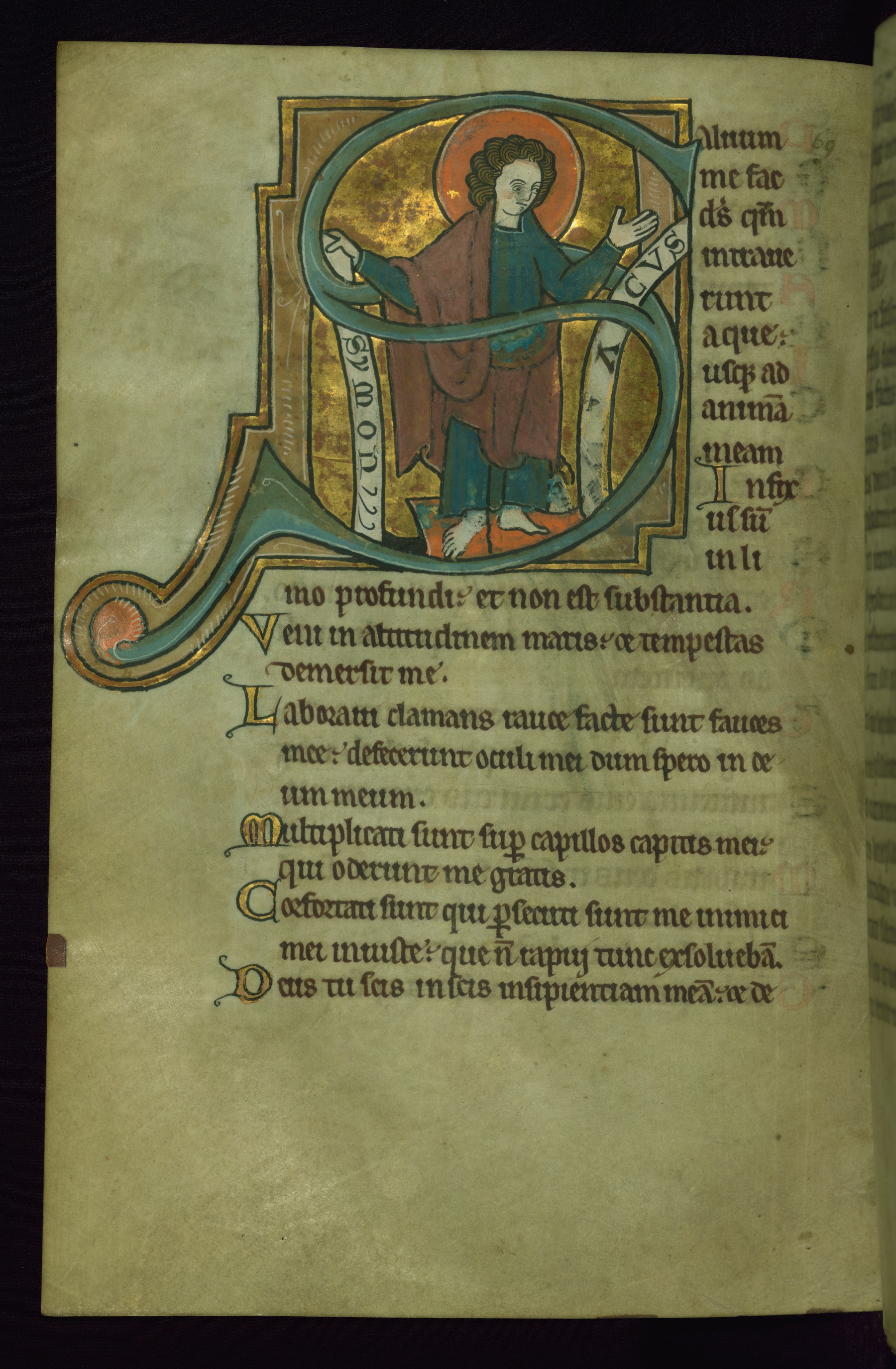This is a detailed color photograph of a page from a medieval manuscript, possibly inscribed in Latin. The page is richly decorated, featuring an ornate, bluish letter "S" that dominates the top left corner. This S is artistically integrated into the image of a person in a manner reminiscent of stained glass artistry. The person depicted is adorned in blue clothing with a maroon robe draped over their shoulder, sporting curly brown hair and bare feet. An orange halo encircles the person's head, suggesting a religious figure. The person is looking downward and to the right. Each sentence of the text begins with an illuminated gold letter, further indicating the manuscript's historical significance. The parchment paper appears old and worn, yet preserved in good condition. The overall colors of the illustration are dark and muted, which complements the ancient feel of the page. This detailed and historically rich illustration and text suggest that it is a page from an ancient religious or scholarly work.